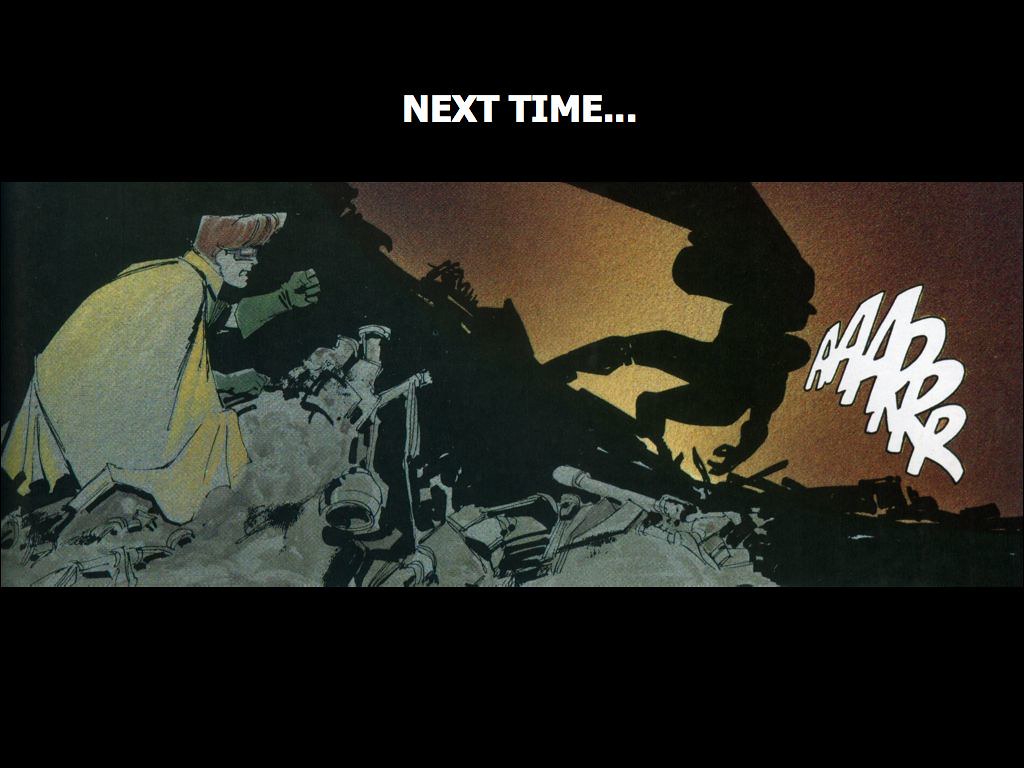This image, possibly a screenshot from a video game or an animated cartoon, features a dark and chaotic scene framed by thick black borders on the top and bottom. In the center, amidst the rubble of what appears to be a war-torn city, stands a character reminiscent of a superhero, drawing visual parallels to Robin from Batman and Robin. This character sports a distinctive flat-top hairstyle, silver glasses, a white cape, and green gloves. He appears to be perched on or near a fallen soldier with a gun, whose silhouette is hard to distinguish due to the dark and fragmented background.

To the right side of the image, emerging from the shadows, is the menacing silhouette of a large monstrous figure, advancing towards the superhero. This monstrous figure is partially obscured, exuding an aura of threat and destruction, and is accompanied by the text "R-A-A-A-R-R-R" in white. At the top of the image, the words "Next time..." are displayed, suggesting a cliffhanger or a continuation of an ongoing narrative. The overall ambiance is one of tension and impending confrontation, set against a backdrop of darkness and destruction.